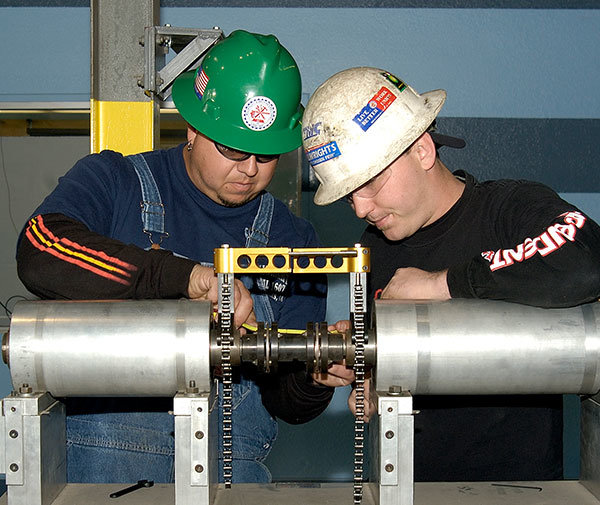The image captures a detailed scene within a construction area or factory environment, where two men, both equipped with safety glasses and different colored hard hats, are engaged in a complex drilling procedure. The background includes a blue wall with varying shades, appearing almost like a garage door with visible metal structures, suggesting an indoor setting.

On the left stands a man named Victor Pat. He is adorned in a green hard hat featuring an American flag and an unspecified logo. Victor is dressed in a blue jumpsuit over a black long-sleeved shirt with striped sleeves, along with suspenders and an earring. He has a prominent beard and a clean hard hat in comparison to his colleague.

To the right, another man, identified as Caucasian due to his pale skin, wears a noticeably dirty white hard hat marked with brown stains and various stickers. He is clad in a plain black long-sleeved shirt. Together, they focus intently on a piece of machinery that includes two cylindrical tubes, a central component with golden and silver hinges, mounted on a gray platform, aiming to fix or assemble it.

The meticulous details of their attire and the machinery illustrate a snapshot of rigorous manual labor in a meticulously organized industrial setting.